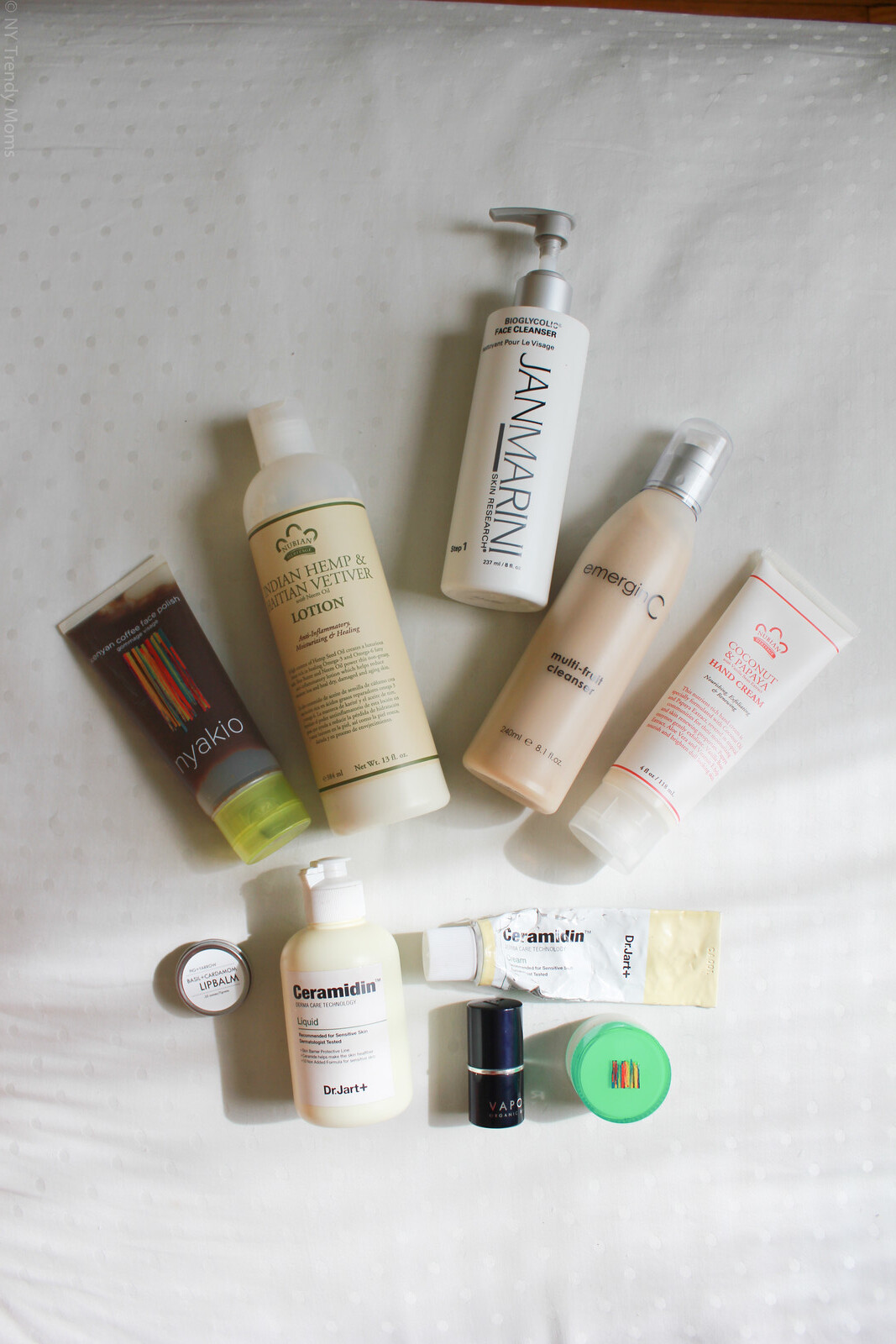This photograph is a vertical overhead shot capturing an aesthetically arranged collection of beauty products. Set against a textured, white surface that resembles a pillow or mattress, the scene is beautifully illuminated by natural light, likely streaming in from a nearby window, casting soft shadows that add depth to the image.

The arrangement features ten beauty product containers evenly divided into two groups: five on the top and five on the bottom. The products are meticulously positioned to display their names clearly. Starting from the top left, the first product is labeled "NYAKIO." Next to it are an Indian hemp lotion, a multi-fruit cleanser, a hand cream, and another unidentified item. 

On the bottom row, the standout product is a tube marked "CERAMIDIN," which appears well-used with its metallic tube showing signs of crumpling and flattening. 

Despite some of the items showing signs of regular use, the overall composition suggests that the products were deliberately arranged for the photograph rather than being placed haphazardly in a typical storage location like a medicine cabinet or a caddy. The careful placement and the interplay of light and shadow create an artful, visually appealing display of everyday beauty essentials.